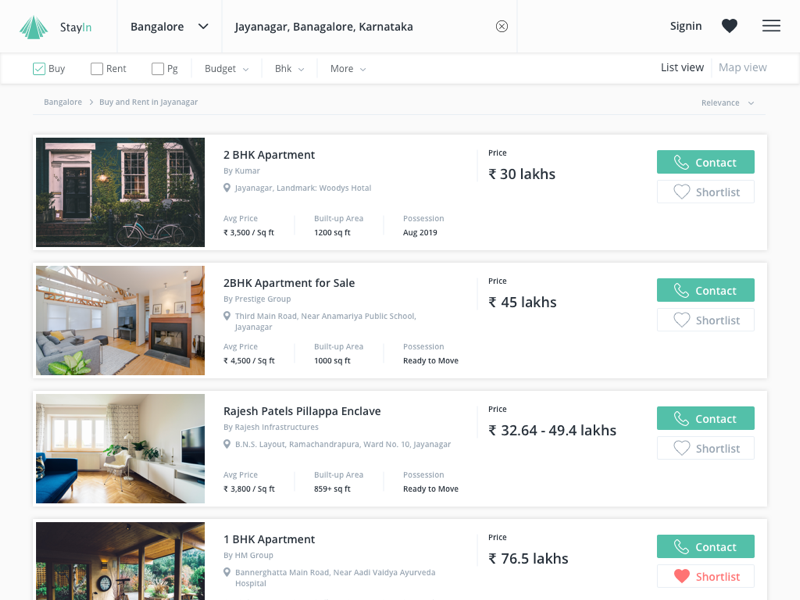The screenshot captures a web page displaying search results for apartments for sale in Bangalore. At the top left corner of the image, there is a green logo accompanied by the word "StayIn" written to its right. Adjacent to this, a drop-down menu labeled "Bangalore" can be seen, followed by the text "Jayanagar, Bangalore, Karnataka". Just beneath this header, a horizontal menu bar presents various options such as Buy, Rent, PG, Budget, BHK, and more.

Following the menu bar, the main section showcases the search results comprising four distinct rows. Each row features a thumbnail image on the left side; these images depict either the exterior or interior views of different houses. The topmost image highlights the exterior of a house with a charming white window and door frames, complemented by an arrangement of flowers. Additionally, a gray bicycle is parked in front of this picturesque house.